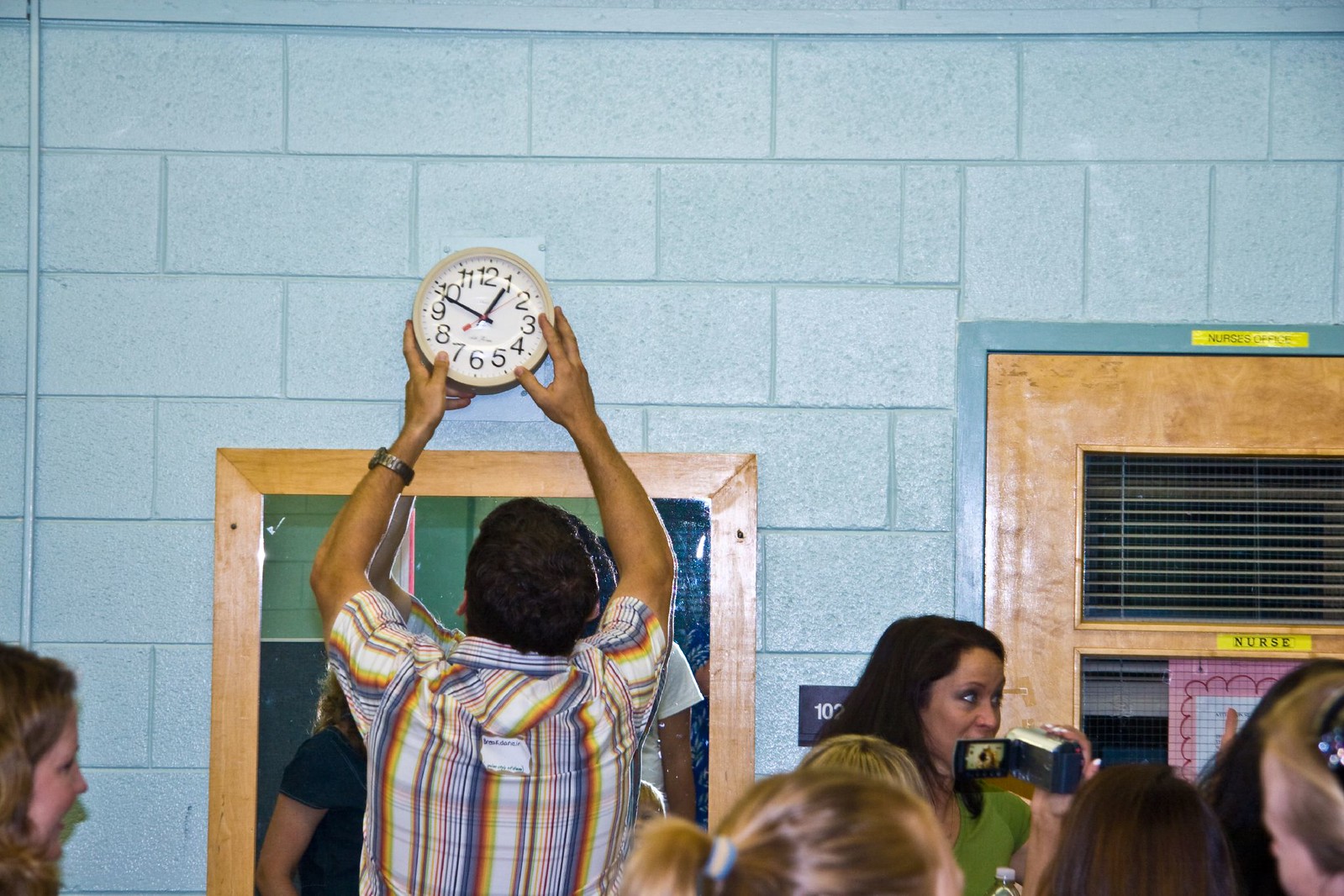In the image, a group of people gather in a room, intently observing a man who is positioning a small, round wall clock on a blue-painted brick wall. The wall is composed of large, stone-like bricks with visible masonry, all uniformly painted in a vivid blue color. The clock is being placed into a square cutout within the wall, which features a flat blue frame, presumably designed to support the clock.

The clock itself is classic and simple, featuring a white border, a white face, black numerals, and black hour and minute hands, along with a red second hand. The man handling the clock is wearing a light-colored t-shirt adorned with vertical stripes in red, yellow, and red. Surrounding him, though less discernible, are several onlookers — women with both light and dark-colored hair, their heads peeking into the frame, adding a sense of group engagement to the scene.